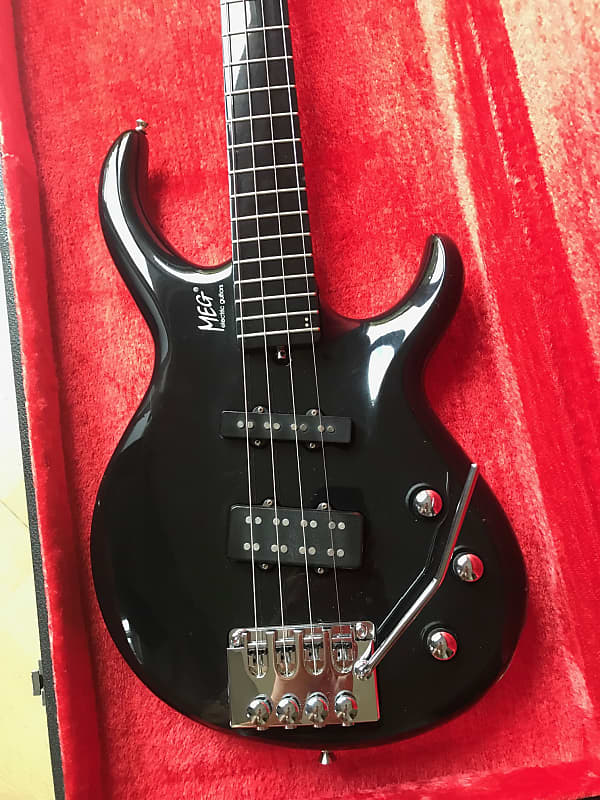This detailed photograph showcases a sleek black electric bass guitar, resting inside an elegant black case lined with plush red velvet fabric. The bass guitar, adorned with the name "MEG" in white lettering near the fingerboard, features a polished body with fancy flame-like cutouts along the top, adding a distinctive flair. The instrument is equipped with chrome accents and fittings, including a metal board that anchors the four strings, a wah-wah bar, and three control knobs. Double pickups are present for enhanced sound versatility, and while there are attachment points for a strap, no strap is included. The photo, taken from above, captures the entire setup with a precision that suggests it might be intended for an online sale, such as on eBay.